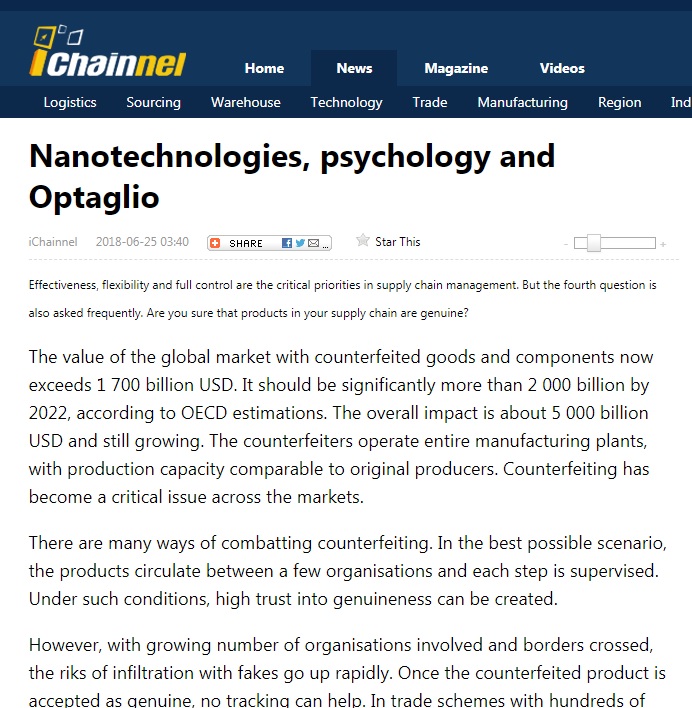The image appears to be a screenshot from a blog or news website named "Chainnail," which seems to be a fusion of the words "channel" and "chain." The website features a clean design with a blue background. At the top left corner, the "Chainnail" logo is prominently displayed in white and yellow. 

To the right of the logo, there is a navigation bar with links labeled "Home," "News," "Menu," and "Videos." Directly beneath this navigation bar is a sub-menu because the "News" section is currently selected. This sub-menu includes categories such as "Logistics," "Sourcing," "Warehouse," "Technology," "Trade," "Manufacturing," "Region," and "IND," which is likely short for "Industry" but is partially cut off.

The main content features an article titled "Nanotechnology, Psychology, and Optaglio." According to the header, this article was posted on "iChannel" on June 25, 2018, at 3:40 PM. Below this, there are social media sharing buttons, a star button for bookmarking, and a text adjustment slider for better readability.

The article's subtitle emphasizes key priorities in supply chain management: effectiveness, flexibility, and full control. It also raises an important question about product authenticity within the supply chain. The article text follows this subtitle, delving deeper into the topic.